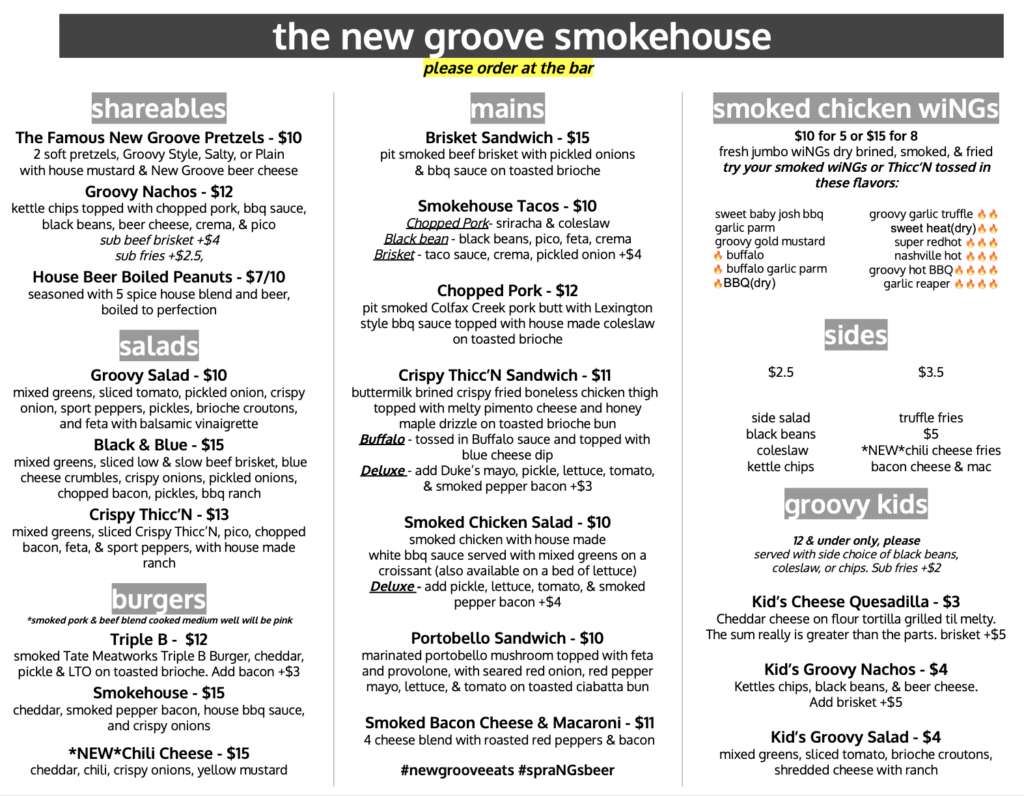This image shows a screen grab of a restaurant menu for "The New Groove Smokehouse." The menu is predominantly styled with black and gray backgrounds and white text. At the top, a long black rectangle features the restaurant's name in white letters: "The New Groove Smokehouse." Directly below this, highlighted in yellow, are the black words "Please order at the bar."

The menu content is organized into three main columns: 
- **Left Column:** This section includes categories for "Shareables," "Salads," and "Burgers," each with a gray background and white text. Detailed descriptions are provided under each category to elaborate on the food items.
- **Middle Column:** Labeled "Mains" in gray and white, this column lists the primary food options, featuring a variety of sandwiches and other main dishes.
- **Right Column:** Begins with "Smoked Chicken Wings," followed by the "Sides" category, and ends with "Groovy Kids," which lists the items available on the kids' menu.

The layout is clean and structured, with distinct separations between each category, making it easy for customers to navigate and choose their meals.